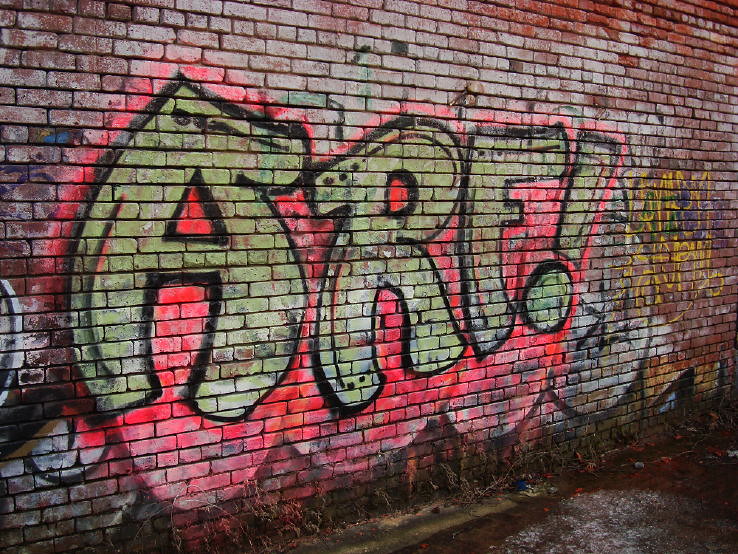The image depicts a section of an old, worn-down brick wall, situated outdoors, with a grimy sidewalk visible at the bottom. The focal point of the photograph is a prominent piece of graffiti that spans the center of the wall, displaying the word "ARF!" in large, green bubble letters with a red, pinkish outline. The letters "A" and "R" feature extensions resembling a head or nose with black dots suggesting eyes. Surrounding this central graffiti, the wall is layered with various other graffiti in yellow, purple, and green paints, indicating that multiple artists have contributed over time. The wall's surface has remnants of numerous past graffiti, now chipped and faded, blending with the multi-colored new additions. The scene includes a bit of overgrown grass and weeds near the base, suggesting it was taken on a damp day.